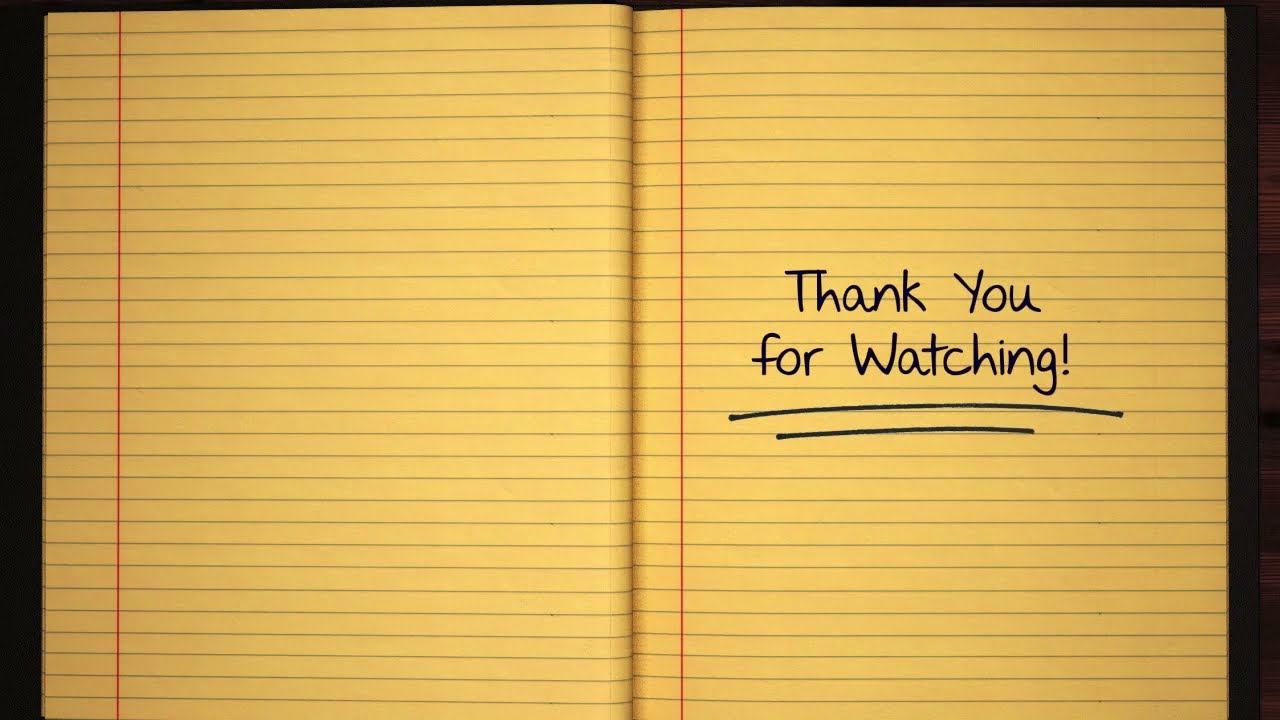This image depicts an open notebook with yellowish loose-leaf paper, featuring a red vertical margin line on the left side and horizontal blue lines for writing. The paper looks like typical lined stationery commonly used in back-to-school notebooks of about 80 to 100 pages, with no visible stains or tears. The notebook lies against a black background. On the right-hand page, centered text in black reads "Thank you for watching," with "Thank you" on the first line and "for watching" on the second, followed by an exclamation mark. This text is underlined twice and appears handwritten, possibly with a Sharpie.